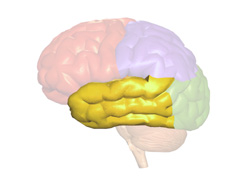The image depicts a highly detailed, computer-generated model of the human brain with different sections color-coordinated. The front area of the brain is overlaid in a transparent, purple hue, while the back top part is shaded in a dark red with a hazy overlay. The right side of the brain showcases a bright, solid yellow mustard color, emphasizing the brain's intricate folds and texture. This yellow section curves from the front middle around the side to the back near the brainstem, forming three folded lines. The overall background of the image is a consistent, clear white, enhancing the bright visibility of the brain's colors and textures.